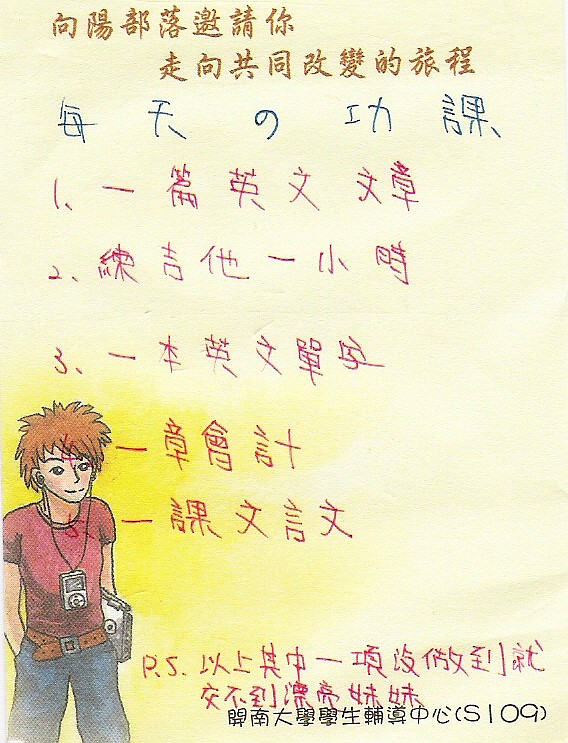In the bottom left corner of the image, there is a cartoon-like illustration of a young person, possibly a teenager, with short, spiky brown hair. The character is wearing a red short-sleeved top, blue jeans, and a brown leather belt. They have a rectangular electronic device, possibly a music player, on their chest with earphones connected and reaching their ears. The character also appears to be carrying a book. The background behind the character is yellow, contrasting with the predominantly pink background of the rest of the page. At the top of the page, there are 11 lines of text written in a foreign language that appears to be Chinese, with the characters written in gold and blue. To the right of the character, there is additional writing, and towards the bottom of the image, the text includes “PS” followed by more Chinese characters.